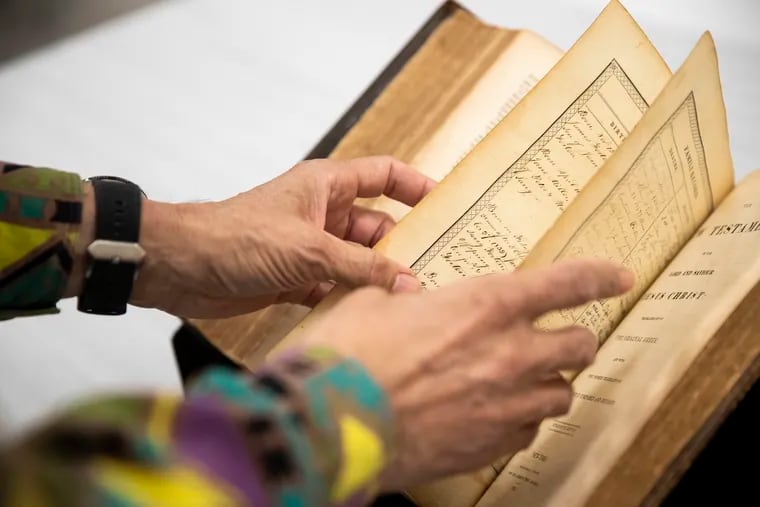This close-up photograph captures an elderly man's tan, hairy hands, mid-turn, rifling through the frail, yellowed pages of an old Bible, which is evident by the discernible printed words "Testament" and "Jesus Christ" on the right-hand page. The man is wearing a black wristwatch on his left wrist, and his vibrant 90's era jacket features bright geometric patterns in neon yellow, purple, and blue. The book's brown leather-bound cover and its seemingly handwritten cursive notes highlight its aged and cherished condition, all set against an out-of-focus white background.